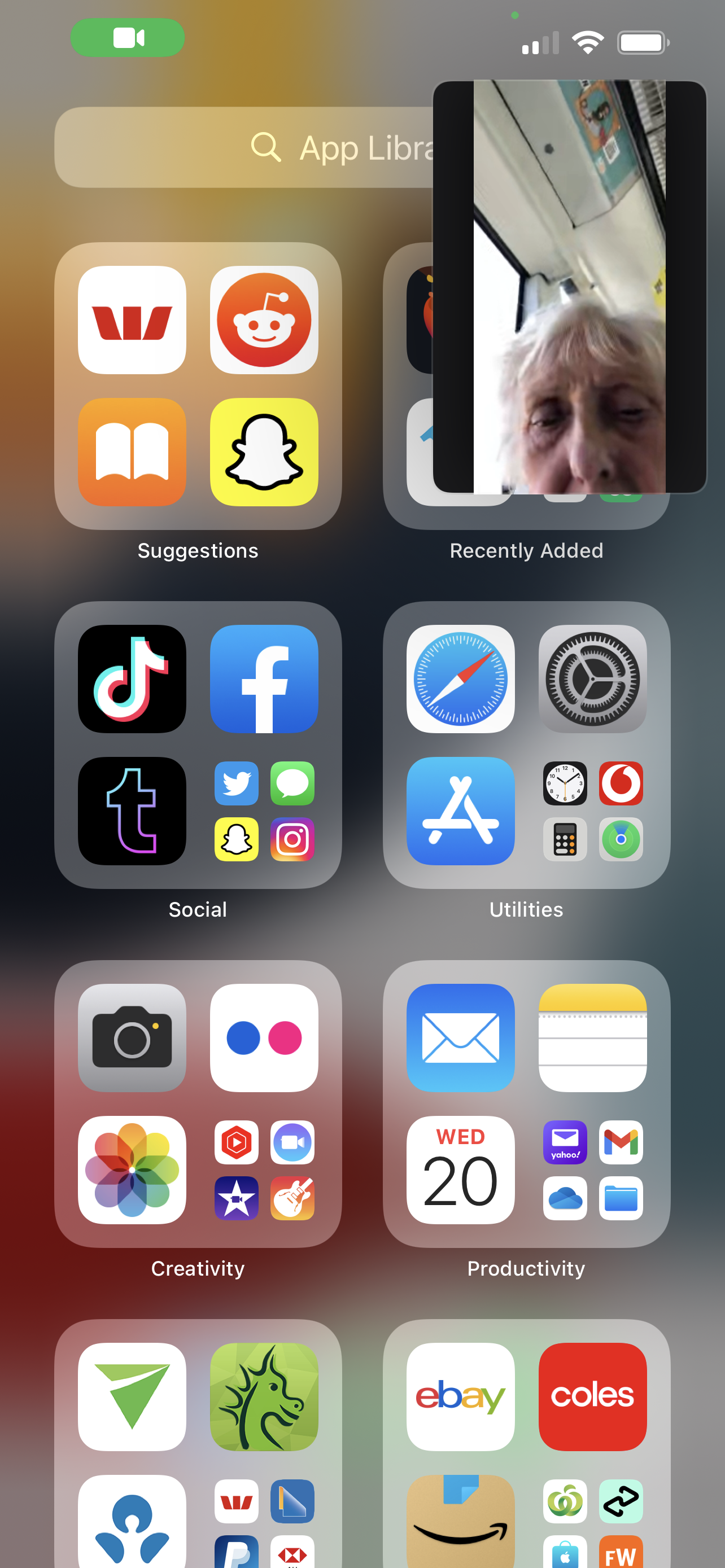This image is a screenshot from a cell phone, featuring various UI elements overlaid on a blurred, gray background. In the top left-hand corner, a green oval contains a white movie camera symbol, signifying a video-related function. The top right-hand corner hosts a set of intricate icons: two vertical lines, followed by three horizontal, curved lines, and a white-filled rectangle, likely indicating different interface options.

The background is predominantly gray and blurred, incorporating darker hues that give it a semi-transparent but almost opaque appearance, allowing a faint glimpse of the underlying image. Central to the screenshot are multiple rows and columns, each consisting of four interconnected smaller squares within a larger gray square. These squares are arranged in a neat grid pattern, with each miniature square showcasing a distinct symbol and color, providing a variety of functions or shortcuts.

Overlaying the top right section is a small, translucent rectangle featuring a person's face, presumably engaged in a video call or conferencing app. The individual appears to be on a train, surrounded by a grayish background with indistinct advertisements visible behind them. The overlay has black bars on either side of it, encapsulating this snapshot of the person's face within the greater complexity of the interface.